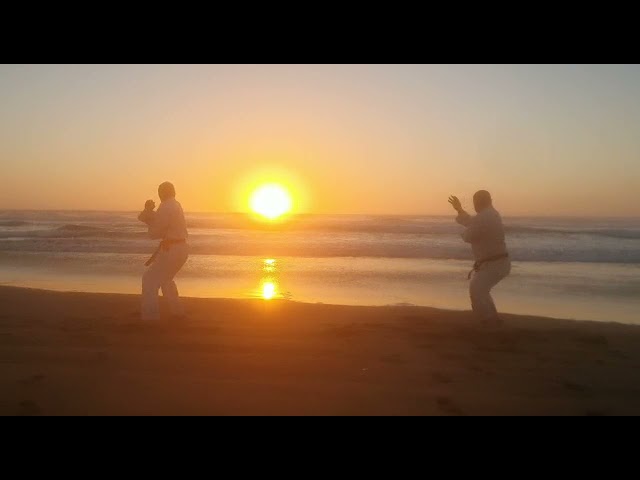The image captures a cinematic scene of two men on a beach, framed in a widescreen format reminiscent of a movie still. The photograph, realistically rendered, shows the men standing on damp sand, facing a calm ocean as the sun either rises or sets, casting a tranquil light across the landscape. The sky transitions through hues of orange, pink, and violet, with a brilliant yellow sun whose reflections shimmer across the light blue-gray water. The men are dressed in traditional white martial arts uniforms complete with belts, suggesting an early morning or evening training session in karate or a similar discipline. Their figures are more silhouetted than detailed, with distinguishable clothing and shapes, yet their specific features remain hidden. They stand in synchronized martial arts stances, legs apart and arms raised in poised gestures. The serene environment, combined with the disciplined postures of the men, evokes a moment of focused practice set against nature’s serene backdrop.